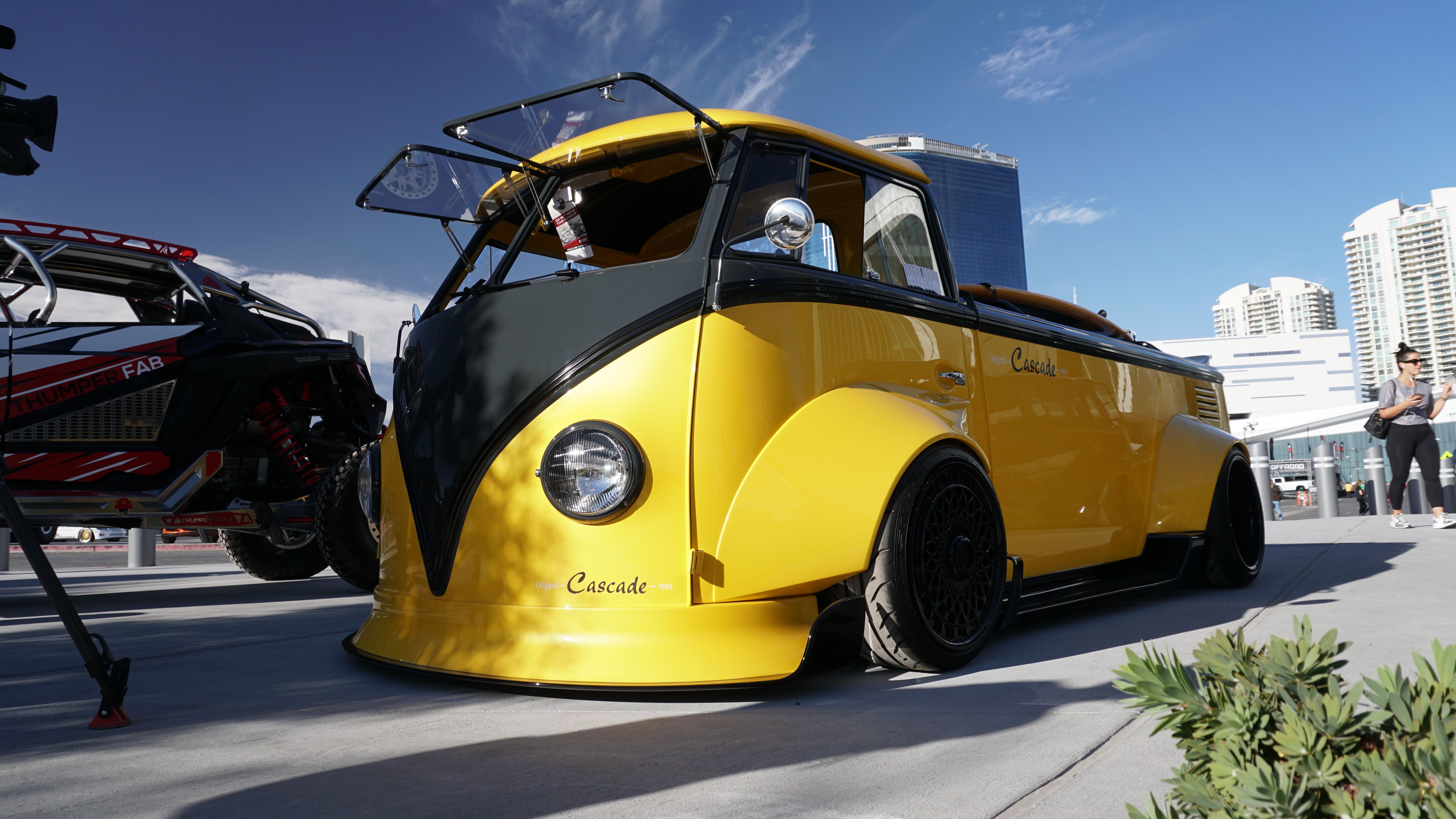In this outdoor photograph, the vivid blue skies dotted with little whiffs of puffy clouds form a serene background. Towering white buildings stand in the right background, while a woman with her hair pulled back, dressed in a gray shirt and dark gray pants, walks nearby. The focal point of the image is a large, futuristic yellow vehicle that stands out with its unique design. This vehicle, labeled "Cascade" on the front, resembles a bus in size but has a roundish, unconventional shape with elements of a truck. The front windshields are split into two sections and opened outward, giving it an open look. The vehicle’s body is predominantly yellow with black detailing, featuring round glass headlights, and pronounced wheel wells over thick black tires. It’s parked on a gray sidewalk or pavement, adding to the urban setting. Beside this striking vehicle is another car, elevated and featuring black, red, and white colors. The scene exudes an impression of a busy city day, possibly during an automobile show, with the futuristic vehicle drawing much attention against the backdrop of a bustling city.